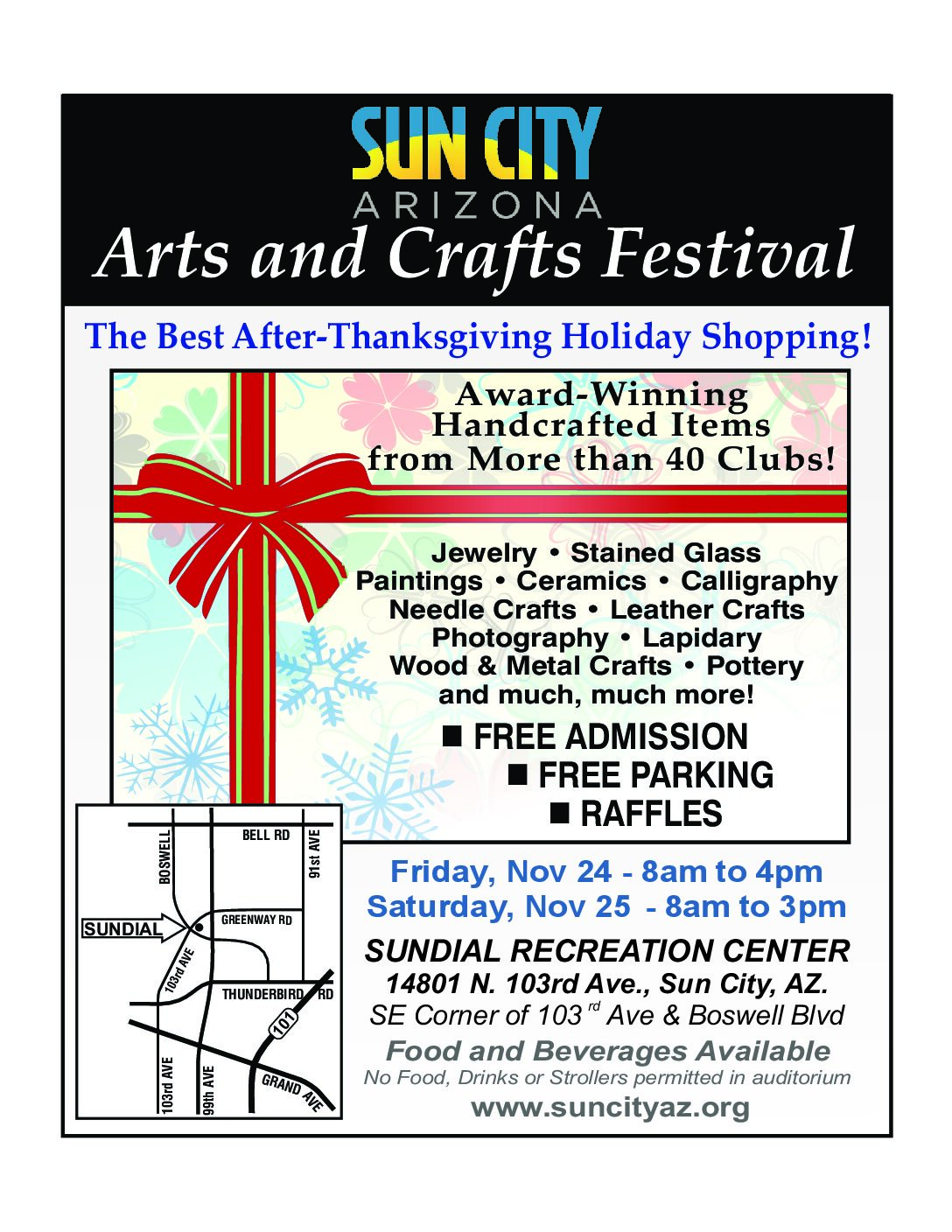This is a detailed poster for the Arts and Crafts Festival in Sun City, Arizona, designed to attract visitors to a post-Thanksgiving holiday shopping event. The poster prominently features Sun City in blue and yellow hues at the top, evoking the sky and sun of Arizona. It advertises the festival scheduled for Friday, November 24, from 8 AM to 4 PM, and Saturday, November 25, from 8 AM to 3 PM, held at the Sundow Recreation Center, 14801 North 103rd Avenue.

The overall design is festive and winter-themed, with a package motif including a red and green ribbon and dotted with snowflakes to capture the Christmas spirit. The poster offers practical information such as free admission, free parking, and details about raffles. There is a small map in the lower left corner to help attendees locate the venue. The middle section features an image of a present tied with a bow, emphasizing the gift-giving season, while a banner at the top proclaims the event's name and purpose. Additionally, the poster highlights the availability of award-winning handcrafted items from more than 40 clubs and mentions the provision of food and beverages.